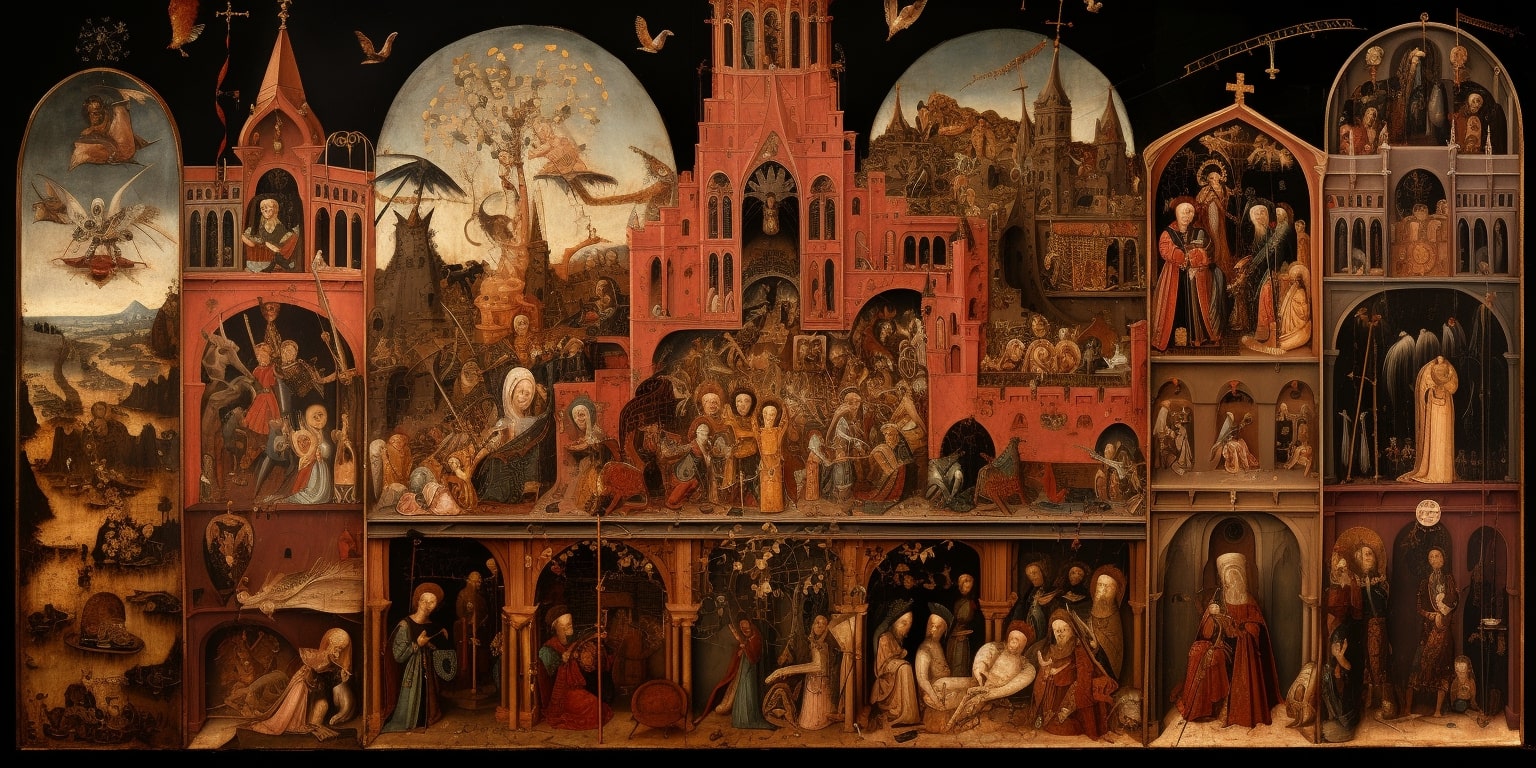This detailed illustration depicts a bustling medieval scene characterized by its religious and mythical elements. Set against a black night sky, the artwork features a large, orange-red building with numerous intricate arches, giving the impression of a church or a religious structure. The building's interior is shown in a cross-section view, revealing multiple rooms where various activities are taking place.

In the foreground, several religious figures, possibly bishops, are prominently featured, highlighted by the presence of numerous crosses. The scene inside the building is lively, with groups of people engaged in a variety of activities such as playing instruments, eating, and observing a lifeless figure. The atmosphere is further accentuated by the building's red spired towers and the predominant use of red hues throughout the painting.

In the background, the mythical undertones are evident with strange flying creatures, including dragons, soaring over a distant castle on a hillside. This medieval painting, likely a piece that could adorn the walls of a church, seamlessly blends the sacred with the fantastical, creating a richly detailed and immersive tableau.